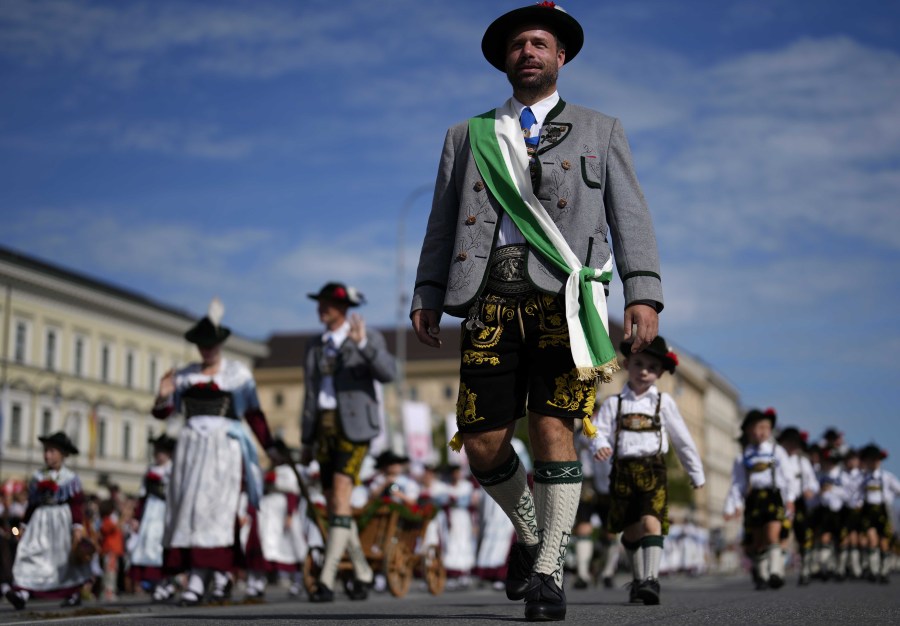This photograph, measuring approximately six inches wide by three inches high, captures an outdoor daytime parade with an emphasis on traditional German attire. At the heart of the image stands a confident man with slightly tanned skin, donning brown Lederhosen adorned with gold embroidery, knee-high gray socks with green tops, and a gray jacket accentuated by a green and white sash. His hat's black brim is visible, though the top is not. He is centrally positioned and in focus, extending a subtle smile.

Surrounding the man, to the right, are schoolboys similarly dressed in Lederhosen, while to the left, men in Lederhosen and women in long skirts paired with white blouses and aprons are visible. The parade takes place in front of impressive, multi-story stone buildings that resemble a royal palace, adding grandeur to the scene. The sky above is a vibrant blue with scattered white clouds, suggesting a sunny day, although the photo appears slightly underexposed, lending it a darker tone overall. The central figure stands out in sharp detail, while the rest of the parade participants are blurred in comparison.